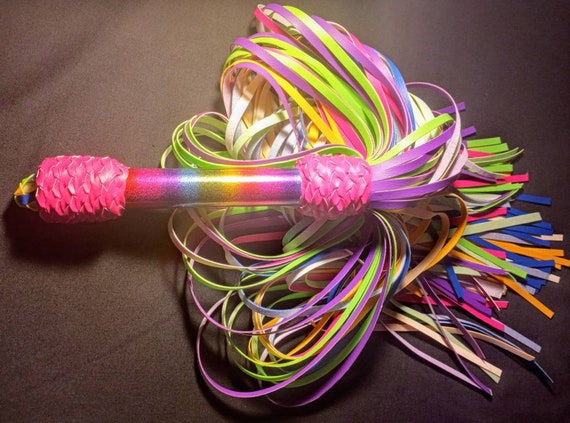This is an image of a short, handheld baton designed to resemble a pom-pom, resting on a brown surface. The handle is crafted from rainbow-colored plastic, featuring shades of red, orange, yellow, green, blue, and purple, though not in any particular order. Each end of the baton handle is capped with pink-tinted tips, adding a distinct flair. Emerging from one end of the baton are numerous tassels, made of flat plastic strips in an array of colors including pink, purple, green, blue, white, and orange. These tassels cascade out in various directions, creating a vibrant and playful appearance reminiscent of the tassels on bicycle handlebars.